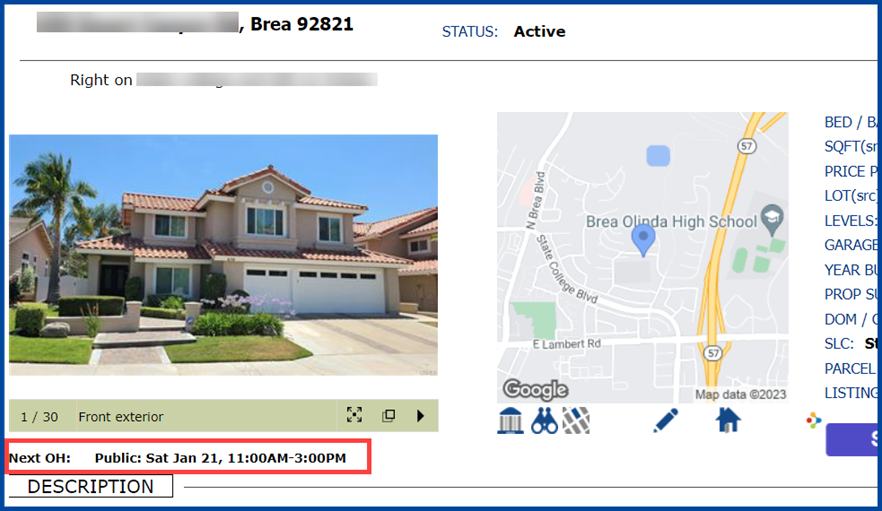The image displays a photograph of a house labeled "Front Exterior." Set against a red outline with bold text, the image indicates an upcoming open house scheduled for Saturday, January 21, from 11 a.m. to 3 p.m. On the right side of the image, there is an embedded Google Maps view showing surrounding roads, including E Lambert Road and State College Boulevard. The map also highlights the location of Brea Olinda High School and the nearby yellow-marked Highway 57. Although the address in the upper-left corner of the webpage is blurred for privacy, the visible zip code "92821" confirms the house's location in Brea, California.